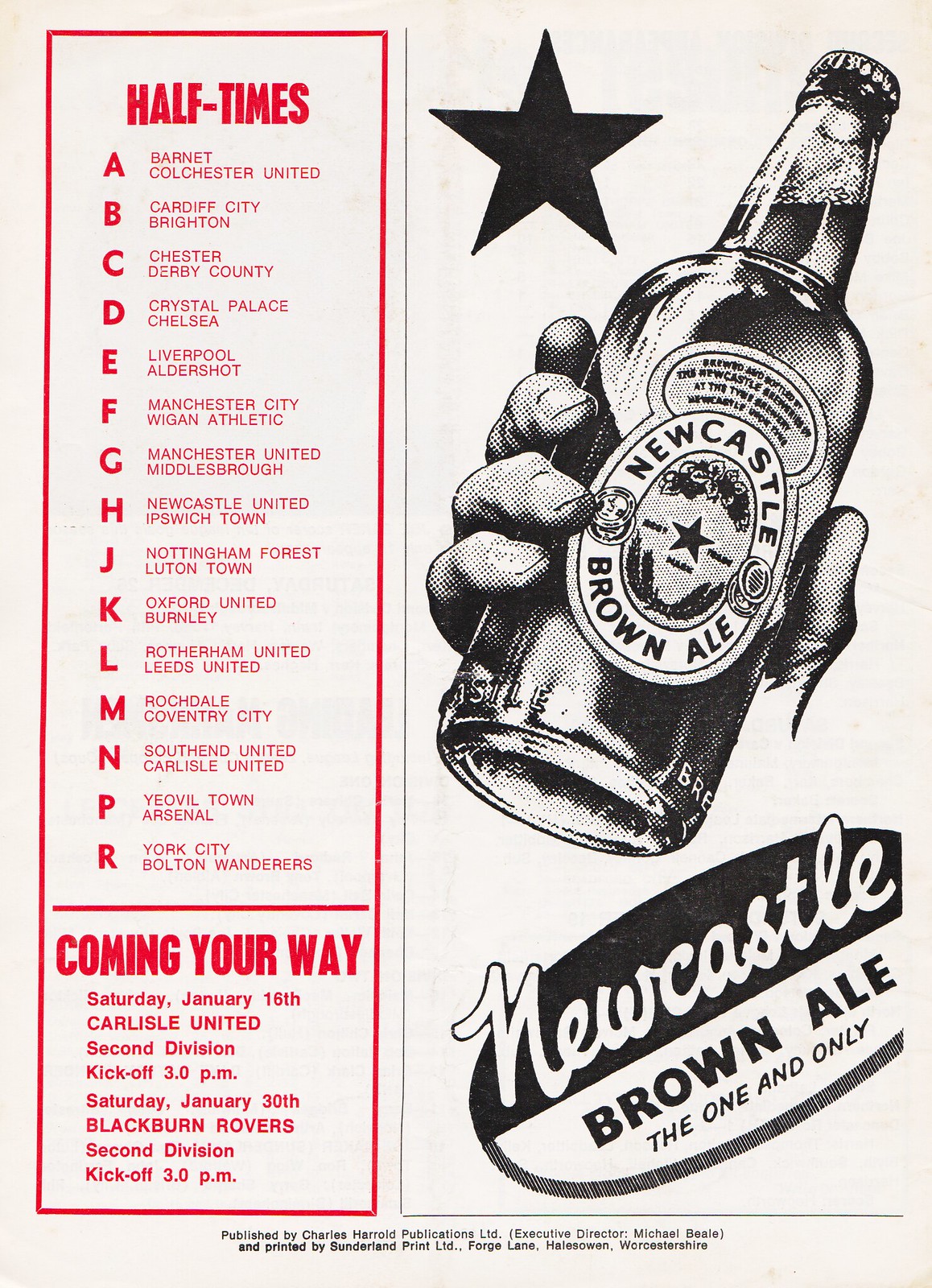This is an intricately detailed vintage advertisement for Newcastle Brown Ale, titled "The One and Only." The ad is split into a red and black color scheme, with the black used for illustrations and the red for text. Dominating the right-hand side, there's a black-and-white sketch of a hand holding a glass bottle of Newcastle Brown Ale, prominently featuring a black star logo. Above the image, the tagline reads "The One and Only" beneath the star.

On the left, a vertical red box is labeled "Half Times" with alphabetical listings from A to R, each associated with different football clubs: Barnett, Colchester United, Cardiff City, Brighton, Chester, Derby County, Crystal Palace, Chelsea, Liverpool, Aldershot, Manchester City, Wigan Athletic, Manchester United, Middlesbrough, Newcastle United, Ipswich Town, Nottingham Forest, Luton Town, Oxford United, Burnley, Rotherham United, Leeds United, Rochdale, Coventry City, Southend United, Carlisle United, Yeovil Town, Arsenal, York City, and Bolton Wanderers.

Beneath the list, also in red, is a highlighted schedule announcement: "Coming Your Way, Saturday January 16th, Carlisle United, 2nd Division, kickoff 3pm," and "Saturday January 30th, Blackburn Rovers, 2nd Division, kickoff 3pm." The advertisement is concluded with fine print noting, "Published by Charles Herald Publications Ltd." and "Executive Director Michael Bill, printed by Sunderland Print Ltd., Porch Lane, Ellesville, Varshastar Shire."